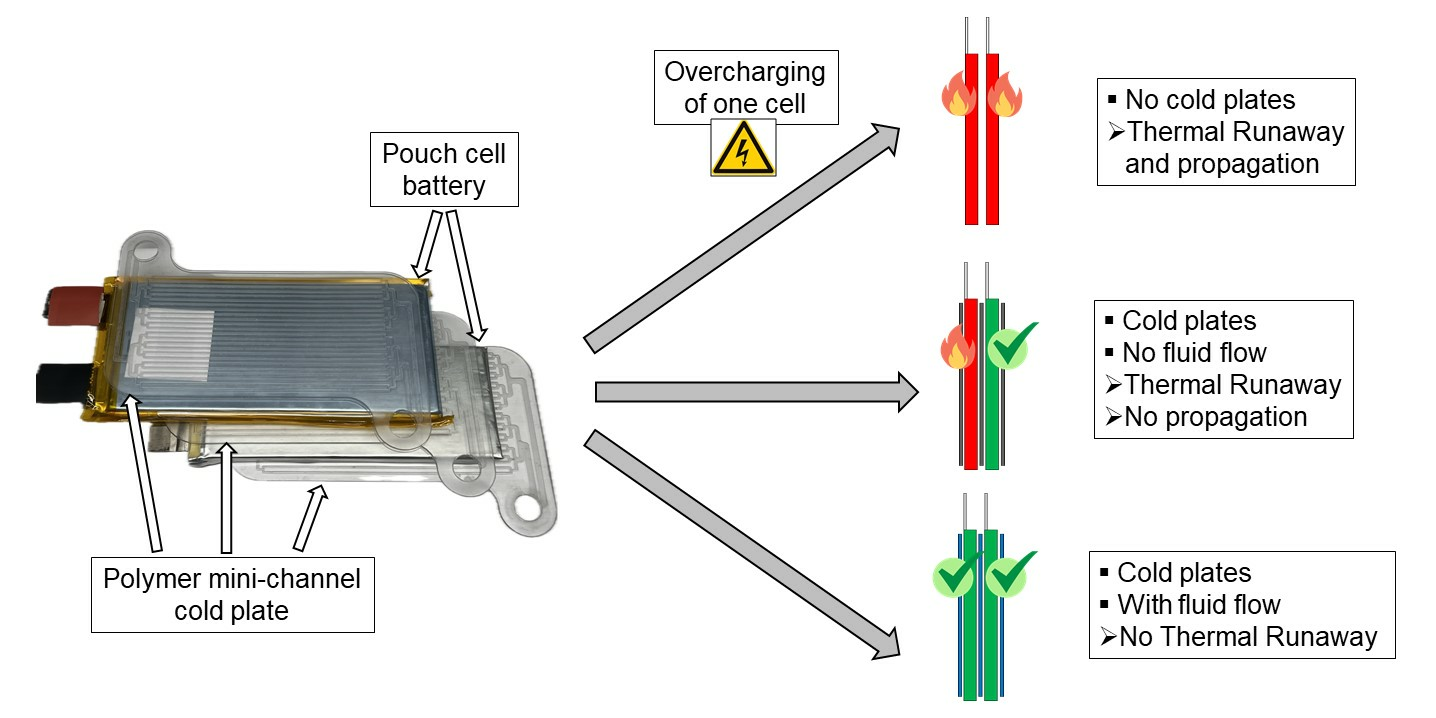This highly detailed diagram illustrates the internal structure and potential thermal behaviors of a battery cell when subjected to overcharging. On the left-hand side, it showcases a disassembled electronic device component, likely a battery, with labeled parts such as "polymer," "mini-channel," and "cold plate." Above, it specifies "pouch cell battery," emphasizing the type of battery in question.

Three distinct arrows depict the outcomes of overcharging one cell, with progressive scenarios from top to bottom:

1. The top arrow indicates a critical failure scenario labeled "no cold plates," leading to thermal runaway and propagation, represented by two red ignited lines.
2. The middle arrow shows a partially mitigated issue, labeled "cold plates, no fluid flow," exhibiting thermal runaway but no propagation, illustrated with a red on-fire section and a green check-marked section.
3. The bottom arrow presents an optimal outcome labeled "cold plates with fluid flow," which prevents thermal runaway entirely, represented by two green lines with check marks.

This diagram serves as an instructional guide on the importance of cooling mechanisms in preventing catastrophic failures during battery overcharging.